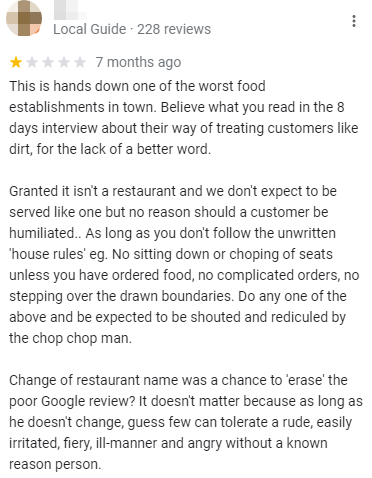This image shows a Google review for an establishment. The reviewer's profile picture and name are blurred for privacy, and they are labeled as a "Local Guide" in gray text to the left. To the right, it lists the number of reviews they have contributed, which is 220. The review is dated seven months ago and the user gives the establishment a 1-star rating, indicated by one yellow star and four gray stars.

At the top right of the review, there is a three-dot settings icon. Below this, the review is broken into three paragraphs, detailing the reviewer's negative experience.

The first paragraph criticizes the establishment as one of the worst in town, mentioning a review from another source that describes poor customer treatment. The reviewer emphasizes that the establishment degrades its customers.

The second paragraph concedes that although the place is not a full-fledged restaurant and thus not all traditional restaurant services are expected, customers still should not be treated poorly. The reviewer lists "unwritten house rules" that seem irrational, such as no sitting down in certain areas, no chopping up seasoned food, avoiding complicated orders, and not crossing specific boundaries.

In the third paragraph, the reviewer notes that even a change in the restaurant's name cannot erase its problematic reputation. As long as the management remains unchanged, the reviewer believes that the negative experience will persist. They conclude on a strong note, expressing their anger and frustration toward the establishment.

Overall, the review paints a picture of a deeply unsatisfactory experience, driven by poor customer service and unreasonable rules.